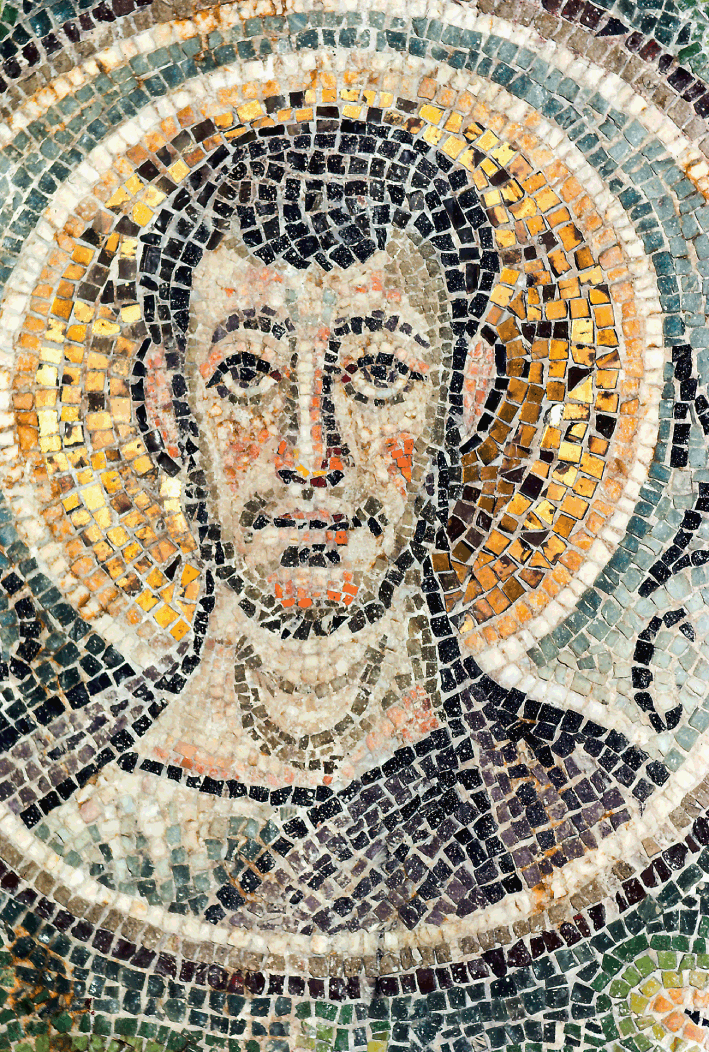This vertically aligned rectangular mosaic art piece features a religious figure composed of an intricate arrangement of small mosaic tiles in various colors, including white, orange, black, and shades of brown and green. The central focus is the face and upper torso of a man, identifiable by his black eyebrows, eyelids, and eyes. His face is tan with distinctive orange spots, a black-outlined mouth edged with brown, and a touch of black under his chin suggesting hair. His head, outlined in black with black squares depicting hair on his forehead, is encircled by a mosaic halo crafted from concentric circles in teal, sage, white, brown, and yellow, with a white outer border. His upper body extends slightly downwards, showing his shoulders and chest shaded in black. The background and the area surrounding the halo feature various colored tiles, enhancing the religious and artistic essence of the mosaic. The craftsmanship and arrangement of these tiny stones give the appearance of a piece that could adorn a sidewalk in a public space or be displayed in a museum.